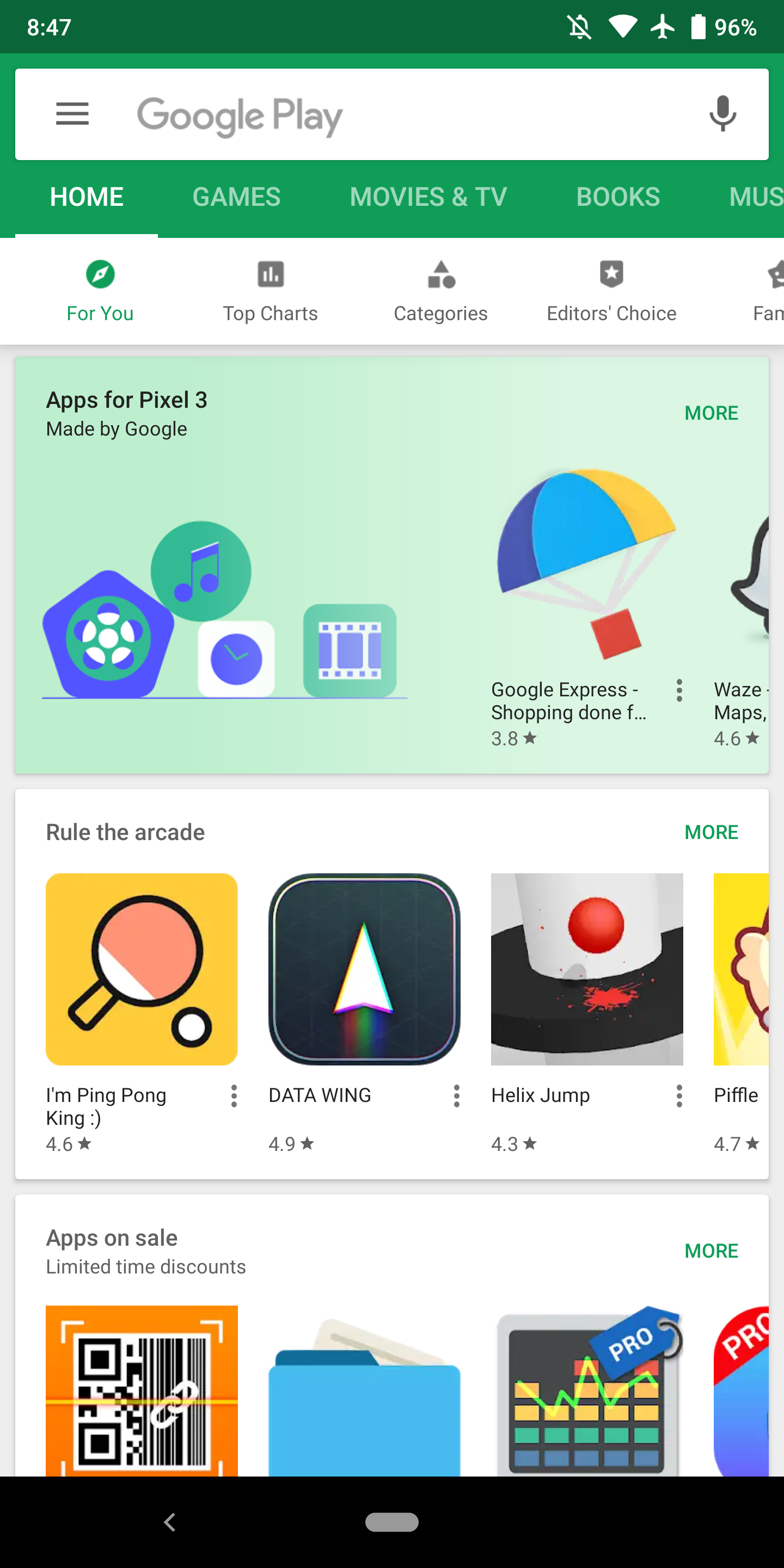This image is a detailed screenshot of the Google Play Store displayed on an Android device. At the top of the interface, there's a green header featuring the Google Play logo. Below it, a horizontal navigation bar includes tabs labeled Home, Games, Movies & TV, Books, and Music. Another row of sub-tabs is visible beneath these, showing options such as For You, Top Charts, Categories, Editor's Choice, and an additional tab partially off-screen.

The interface follows Google's Material Design guidelines, providing a clean and structured layout. Three distinct content sections are visible in the screenshot. The first section, titled "Apps for Pixel 3," features a light green background and highlights a selection of apps promoted for the Pixel 3 phone. It includes a prominent Google Express app recommendation and a green "More" button for additional options.

The second section is titled "Rule the Arcade" and is devoted to arcade-style games. Displayed titles include "I'm Ping Pong King," "Data Wing," and "Helix Jump," with a "More" button for extended browsing.

The final section, titled "Apps on Sale," offers "Limited Time Discounts" on various applications. All visible sections provide a user-friendly interface for browsing and downloading apps, emphasizing Google's cohesive and vibrant design language.